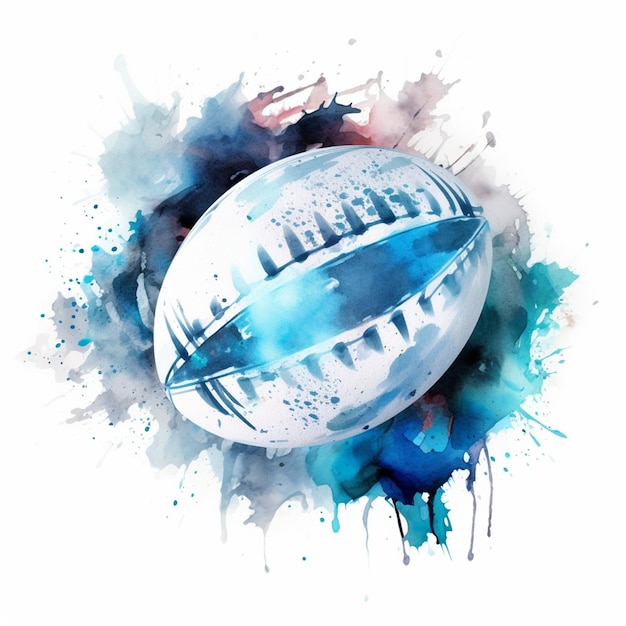The image is a watercolor painting featuring a central object that resembles a whitish rugby ball or football. This object appears to be split open in the middle, reminiscent of an eyelid closing. The inside of the split reveals varying shades of blue, transitioning between light and dark hues. The outer surface is primarily white, accentuated with blue lines and what seem like laces on either side of the split. The background is an all-white canvas adorned with splotches and splashes of color, including blues, pinks, purples, black, and grays. The bottom edge of the painting is characterized by drips of paint, adding to its vibrant and dynamic nature.